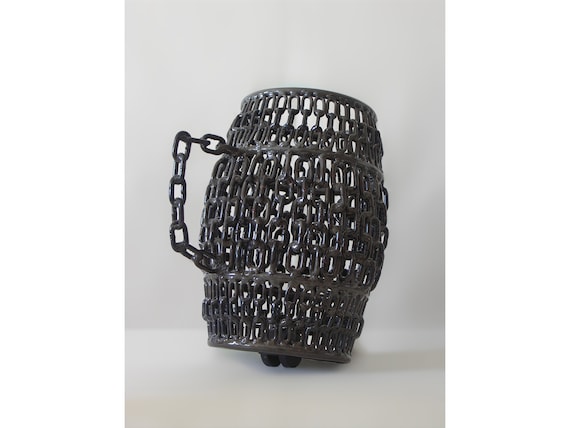The image features an intricately designed tankard with a rounded body and a handle, entirely composed of black cast-iron chain links. The chain links interlock to form the mug, with noticeable gaps between them, and exhibit a glossy black finish. The handle, constructed from single chain links, extends out in a square shape, seemingly defying gravity. The tankard is positioned at an angle, slightly tilted away from the viewer, and appears to be propped up by some form of support at the bottom. Despite a shadow cast to the right, the lack of alignment with the tilt of the object and the indistinct, fuzzy light gray background suggest the image may be AI-generated. The overall scene, set on a white table, showcases the unique craftsmanship and surreal quality of the object.